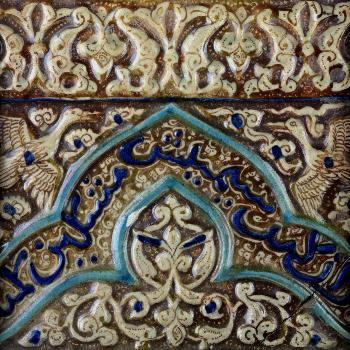The image showcases a highly intricate and ornate tile design that seems to depict a portion of wall or pottery with a strong Mediterranean or Middle Eastern influence. Dominating the foreground is an exquisite tile that appears to almost form the figure of a person, accentuated by light blue outlines and detailed patterns resembling flowers and intertwined vines. These elements converge to create a face-like impression with striking blue eyes. Above this central tile is an array of tiles featuring dark blue script, likely Arabic, which is framed by a harmonious light blue border.

Further up, the design transitions into a depiction of flying ducks and delicate butterflies, rendered in a light beige hue with subtle blue accents. The overall composition is rich with filigree and floral motifs, adding to the sense of historical and cultural depth. Integral to the design are images of birds resembling storks or other waterfowl, enhancing the natural and serene aesthetic of the artwork. The background presents a dark beige tone contrasted against glossy white carvings, which are meticulously detailed and painted.

This visually compelling imagery evokes a sense of timeless beauty and craftsmanship, indicative of a wall in an ancient Middle Eastern or Mediterranean setting, adorned with elaborate, symbolic tiles and script.